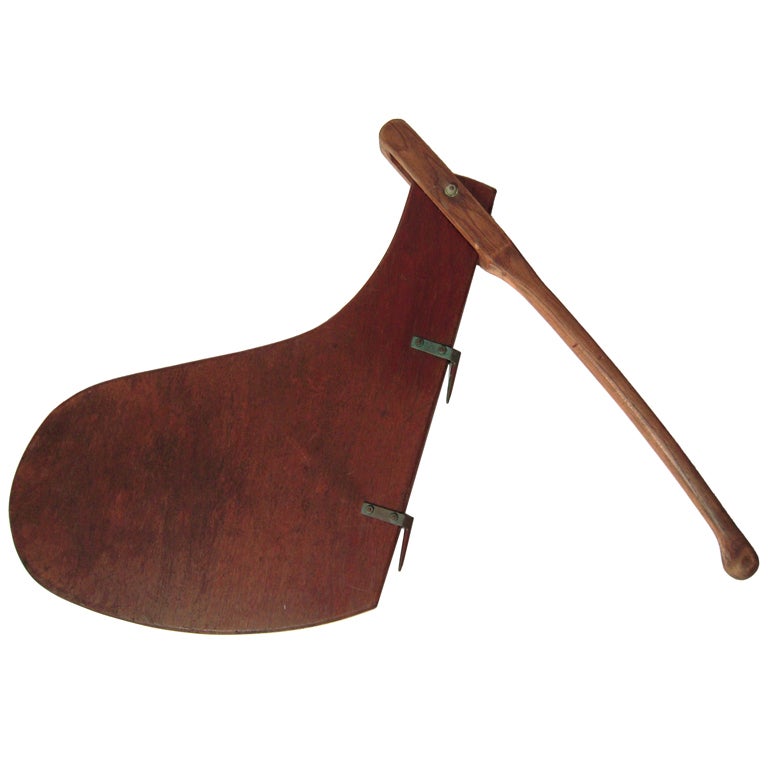On a stark white background, there is a photograph of a peculiar, rustic wooden object, predominantly featuring a rich, reddish-brown mahogany color. The main body of the object is oddly shaped, resembling an ankle and foot or even a filled-in letter 'P'. Affixed to this body are two metallic, gray fasteners positioned on the right side, which seem to serve as attachments, possibly for securing or pivoting another component. Extending from this setup is a more naturally colored wooden stick, rounded and seemingly ergonomic for handholding. This stick is attached to the thinner 'ankle' edge of the main body with a pin or brad, which allows it to pivot, suggesting a functional purpose for the entire assembly. Despite its unclear function, the object appears to be some sort of tool, characterized by its rustic and roughly finished appearance.